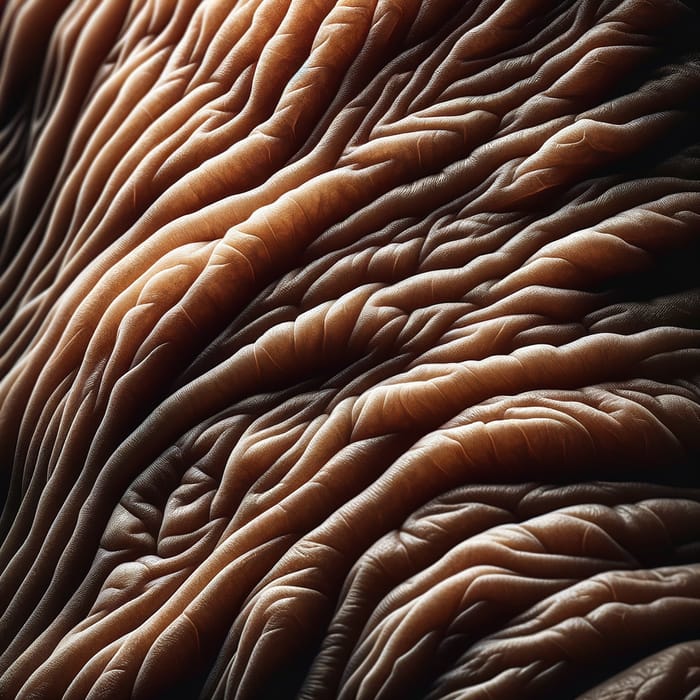This close-up image, likely taken under a microscope or digitally generated, vividly portrays a magnified view of undulating, ridged, and folded skin. The image is dominated by shades of dark pink, purple, tan, and brown, highlighted by a light source from the upper left, creating a dramatic play of shadows. The intricate details resemble the complex, rumpled texture of a mucus membrane or possibly internal body tissues, such as the inside of a nose or ear. The ridges run diagonally from the top left to the bottom right, contributing to the image's abstract, yet slightly unsettling, design, reminiscent of a topographical landscape. The photograph’s emphasis on texture and color contrast highlights its artistic qualities, making it both fascinating and uncomfortable to the viewer.